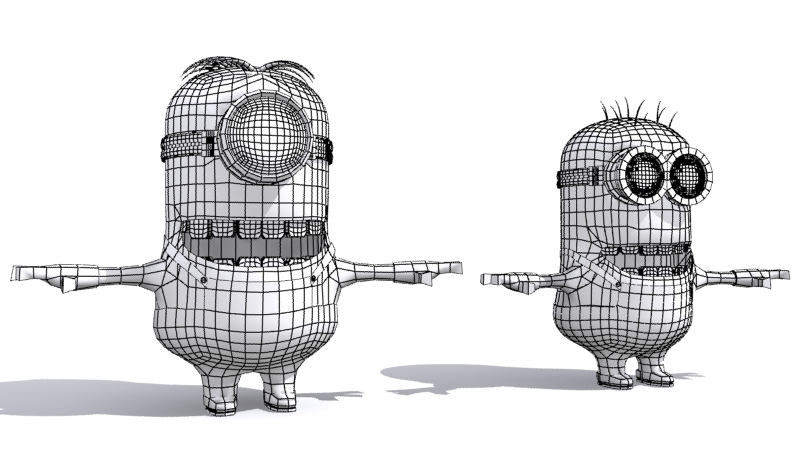This black-and-white digital rendering features two cartoonish characters reminiscent of minions, each casting noticeable gray shadows against a solid white backdrop. The character on the left has a pill-like, oval shape adorned with vertical and horizontal stripes, resembling a fence pattern. This character has a single goggle covering its one eye, a wide open mouth with visible teeth, and tufts of hair sprouting irregularly from its head. It stands with its nubby feet apart and arms outstretched at shoulder level. The counterpart to the right, similar in overall shape, differs by wearing goggles with two eyes and exhibiting fewer hair specks. It mimics the same posture with outstretched arms and bears a tile-like pattern. Their combined stance and detailed textures create a cohesive and professionally rendered image.